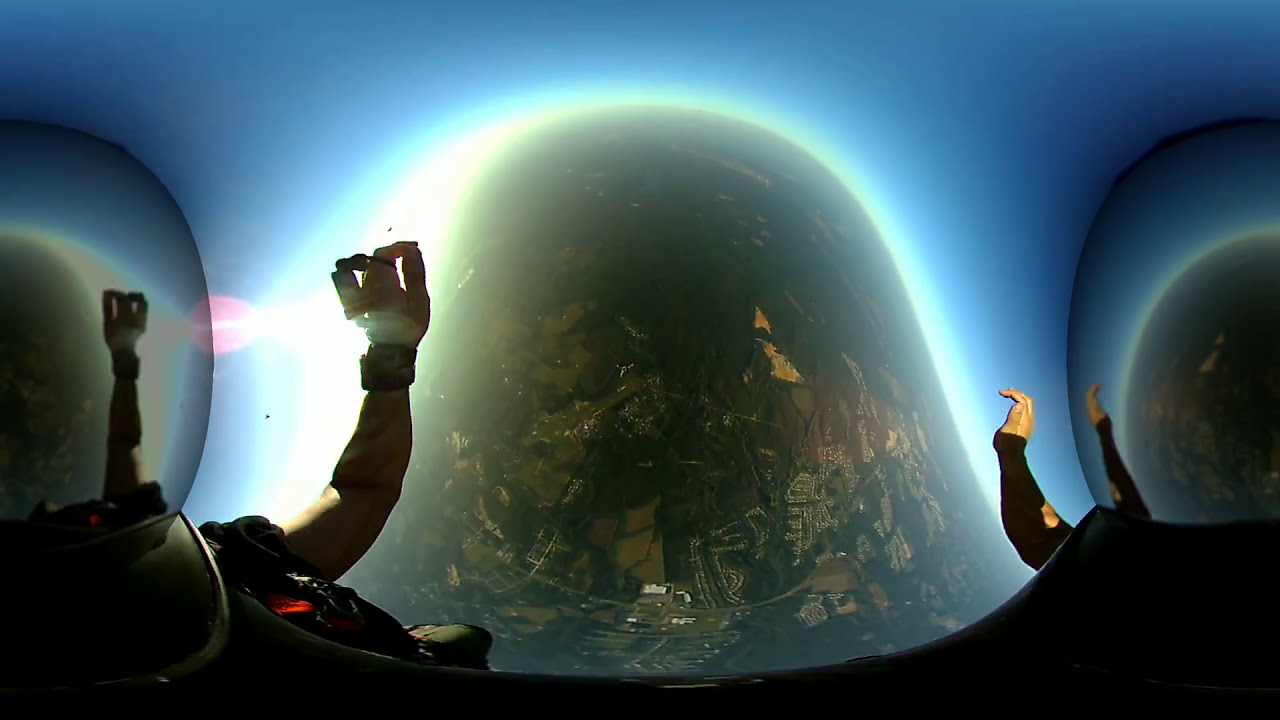The captivating image depicts two skydivers in black vests, poised in the air as they begin their descent from an airplane. Their hands are extended forward, adorned with various instruments likely measuring altitude. Below them, the Earth sprawls with vivid details—roads weaving through patches of green grass, scattered houses, and shimmering bodies of water. The scene, however, has an uncanny twist; the skydivers seem to be floating in a surreal space where the verdant landscape merges with a cosmic backdrop, evoking an almost animated, AI-crafted quality. This unique design further includes an odd blue wall featuring three large, rounded windows that bubble out, contributing a warped perspective to the view. The middle window offers a direct look at the ground far below, enhancing the dream-like, gravity-defying atmosphere. Floating bubbles and hands rising into the frame augment the surreal composition, making it a visually arresting and fresh piece.